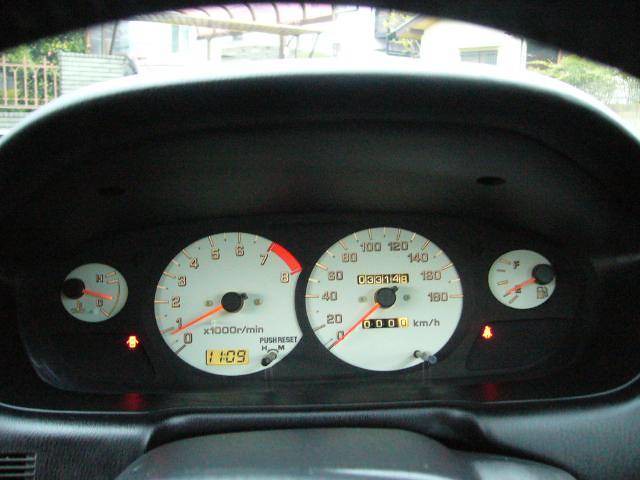A meticulously detailed photograph captures a car dashboard with a striking composition. Dominating the center of the image are four horizontally-aligned dials. The outermost dials on the left and right are considerably smaller, contrasting with the significantly larger inner dials. The right dial slightly overlaps the left inner dial, adding depth to the arrangement. Each dial features a white base with elegant rose gold numbers, and they all have a small black circle at the center with a long red needle pointing to the current reading.

At the bottom left and bottom right of the dashboard, two illuminated indicators are visible. The left one is an orange light signifying an open door, while the right one indicates an unfastened seat belt. These dials and indicators sit within a large, round, dark rectangular panel made of a mostly matte black hard plastic material.

At the top of the image, flanked by the steering wheel on both the left and right, a portion of the car window is visible. The bright, slightly overexposed window reveals a glimpse of a wall, a bit of a garden, and possibly a building. Adding to the complexity of the composition, the bottom section includes a large protrusion, likely the base of the steering wheel. Notably, the middle-left dial displays the text "1109" on a small screen at its base. This photograph exquisitely details the elegant and functional design of the car's dashboard.